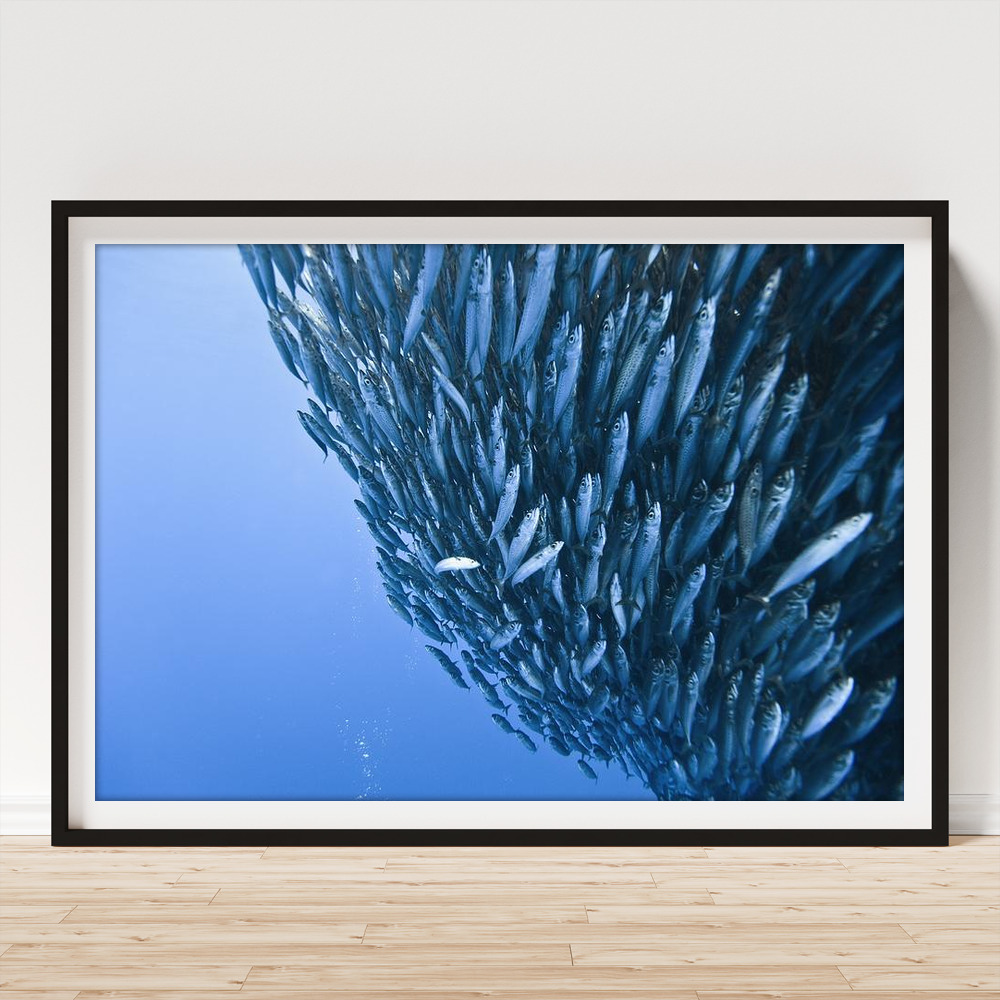The picture features a large painting, captured in a photograph. The painting, encased in a prominent black frame with a substantial white mat, rests on a wooden floor against a stark white wall with a visible baseboard. The painting, measuring approximately four feet by two feet but shown lying on its side, depicts a dynamic underwater scene. A school of fish, possibly consisting of different shades of white, light blue, and dark blue, densely populate the canvas, predominantly occupying the lower right. These fish create a striking contrast against the gradient blue ocean background that spans from light to dark, with a more open expanse on the upper left, forming a diagonal line through the scene. The intricate depiction of the fish in mid-swim encapsulates the movement and urgency of a tightly-knit underwater surge, framing an evocative and lively marine tableau.